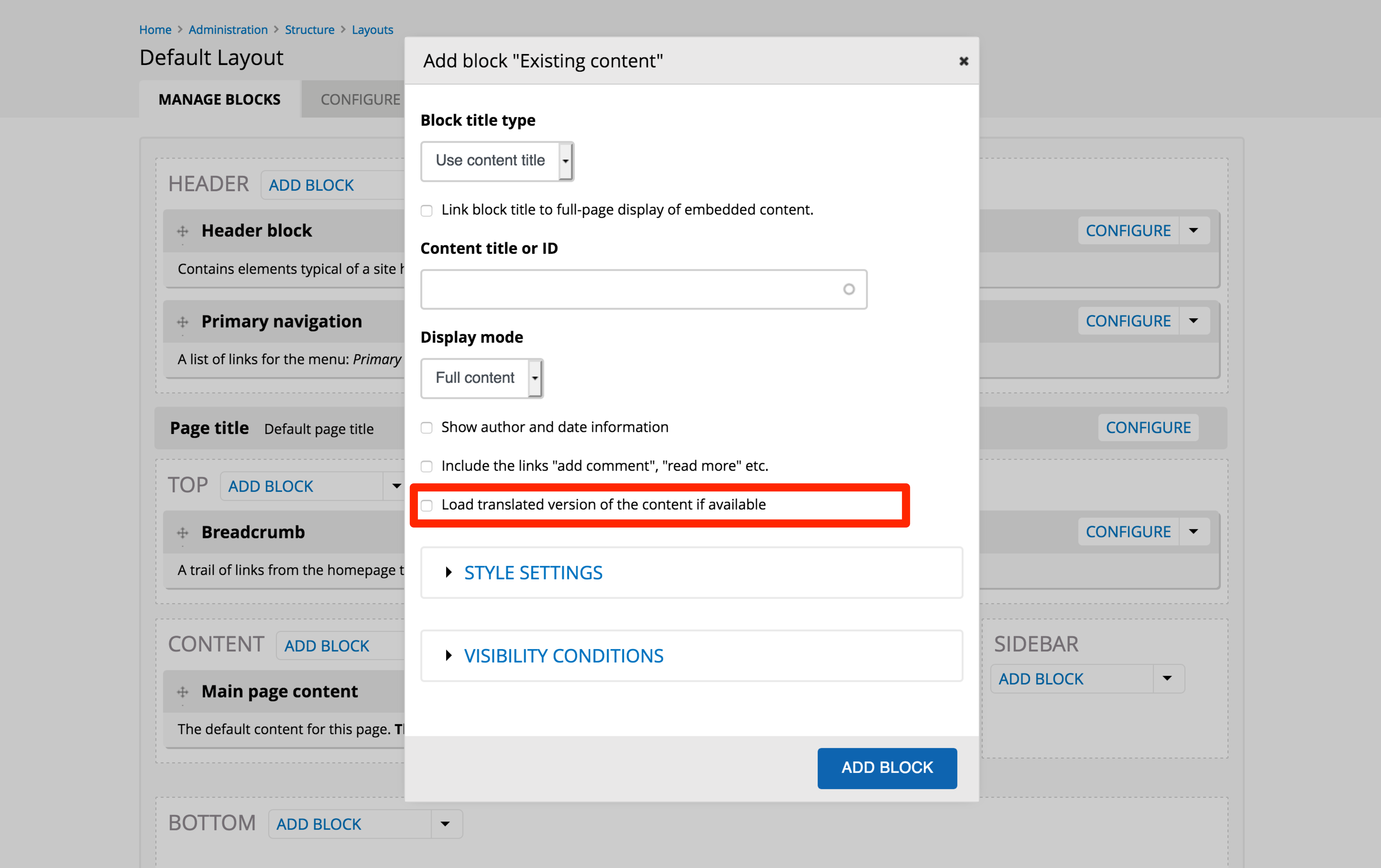The image depicts a screenshot of a webpage featuring a pop-up overlay. The background webpage is grayed out to emphasize the foreground pop-up. The pop-up has a gray header and footer, each providing functionality and instructional elements. 

At the top right corner, there is a black 'X' button for closing the pop-up. The header section indicates the pop-up's purpose, titled "Add Block Existing Content." 

The footer contains bright blue, rounded-corner buttons with white lettering, labeled "Add Block." 

Within the pop-up, the content is organized into several sections through various form controls and options:

1. **Block Title Section**: 
   - A drop-down box labeled "Type" allows the selection of the block type. 
   - An option to use a content tile title, with an unchecked checkbox.

2. **Box Title Linking**:
   - Below is an unchecked checkbox offering to link the box title to a full page display of embedded content.
   
3. **Content Identification**:
   - A field for entering the content title or ID, accompanied by a grayed-out circle on its right.
   
4. **Display Mode**:
   - A drop-down selection for display modes, defaulting to "Full Content."
   
5. **Additional Information**:
   - An unchecked checkbox labeled "Show Author and Date Information."
   - Another unchecked checkbox with an option to "Include links to ‘Add’ and 'Read More'" with “Add” and “Read More” in quotes. This checkbox is highlighted with a bold red rectangle.
  
6. **Translations**:
   - An unchecked checkbox labeled "Load Translated Versions of Content, if available."
   
7. **Style Settings and Visibility Conditions**:
   - These sections can be expanded or collapsed, indicated by right-facing triangles next to their titles.

The pop-up offers robust functionality for adding and configuring content blocks, reflecting an advanced content management interface.